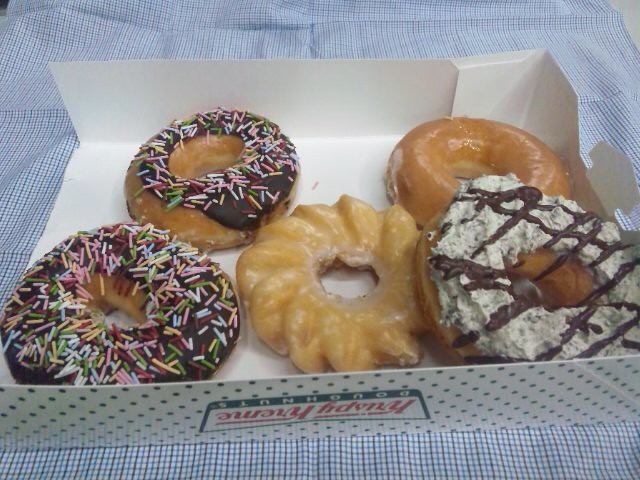This detailed photograph showcases six Krispy Kreme donuts arranged inside a white Krispy Kreme box, which features the brand's iconic logo. The box, identified as the top portion, lies open on a table adorned with a tightly checkered blue and white cloth. The assortment within the box includes two donuts on the left, each with chocolate frosting and pastel rainbow sprinkles. In the center, there is a cruller with a clear, shiny glaze that gives it a yellowish-brown hue. Towards the back right, a plain Krispy Kreme glazed donut shares the same yellowish-brown color as the cruller. Finally, on the bottom right, there is a donut topped with white icing, possibly cookies and cream, accented with a crisscross pattern of chocolate drizzle. The composition and colors offer a visual feast, highlighting the variety and appeal of the donuts against the simple, geometric background.